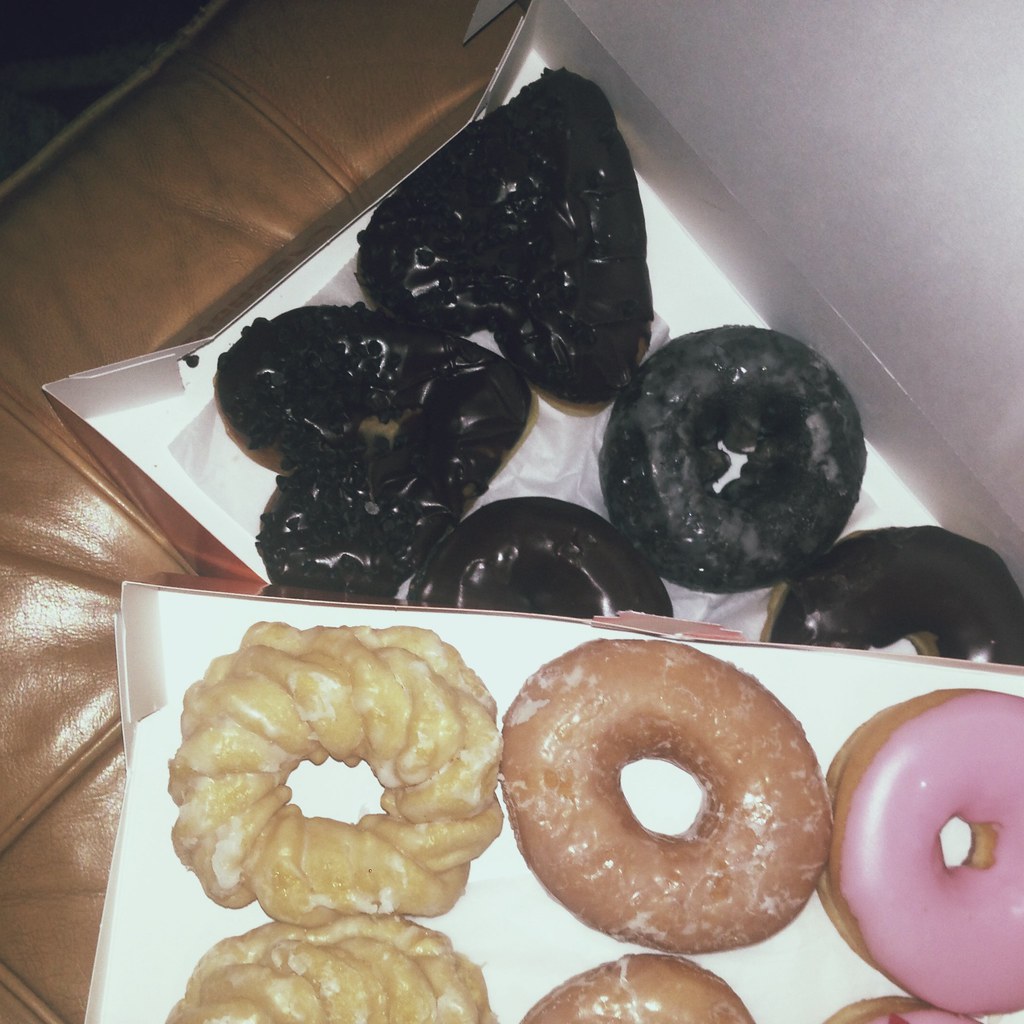This is a top-down image of two white boxes, each containing six donuts, stacked askew on a light brown or tan leather seat cushion or ottoman, possibly within a car or living room setting. The lower box, partially obscured by the top box, houses a collection of dark chocolate or black donuts: four are regular-shaped while two are heart-shaped. In the upper box, which dominates the lower third of the frame, the donuts are arranged in pairs: two braided or rope-shaped crullers with a white glaze, two standard glazed donuts, and two donuts coated in pink frosting without sprinkles. The rich detail of the leather surface behind the boxes adds a warm tone to the setting.